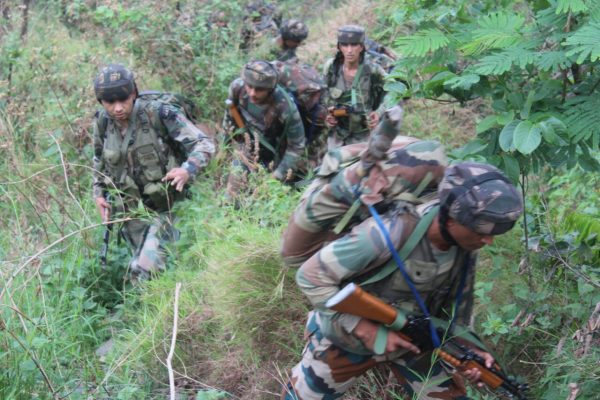In this photograph, a group of soldiers is seen navigating a jungle environment, dominated by hip-high vegetation, including tall grasses, bushes, and brown shrubs. In the foreground, a soldier wearing an olive green camouflage uniform with splotches of darker green, black, brown, and blue stands prominently. He dons a matching camo cap and carries an AK with a wooden stock, pointed down, suggestive of a leading position. His camouflage backpack is slung over his shoulders. Behind him, four more soldiers, similarly attired and armed, follow in formation. They also wear camo outfits and caps, blending with the surrounding flora though still discernible. The scene is set in a clearing amidst tall grasses and sparse trees, bathed in daylight. Further in the background, another group of soldiers can be faintly seen, their figures blurred and distant.